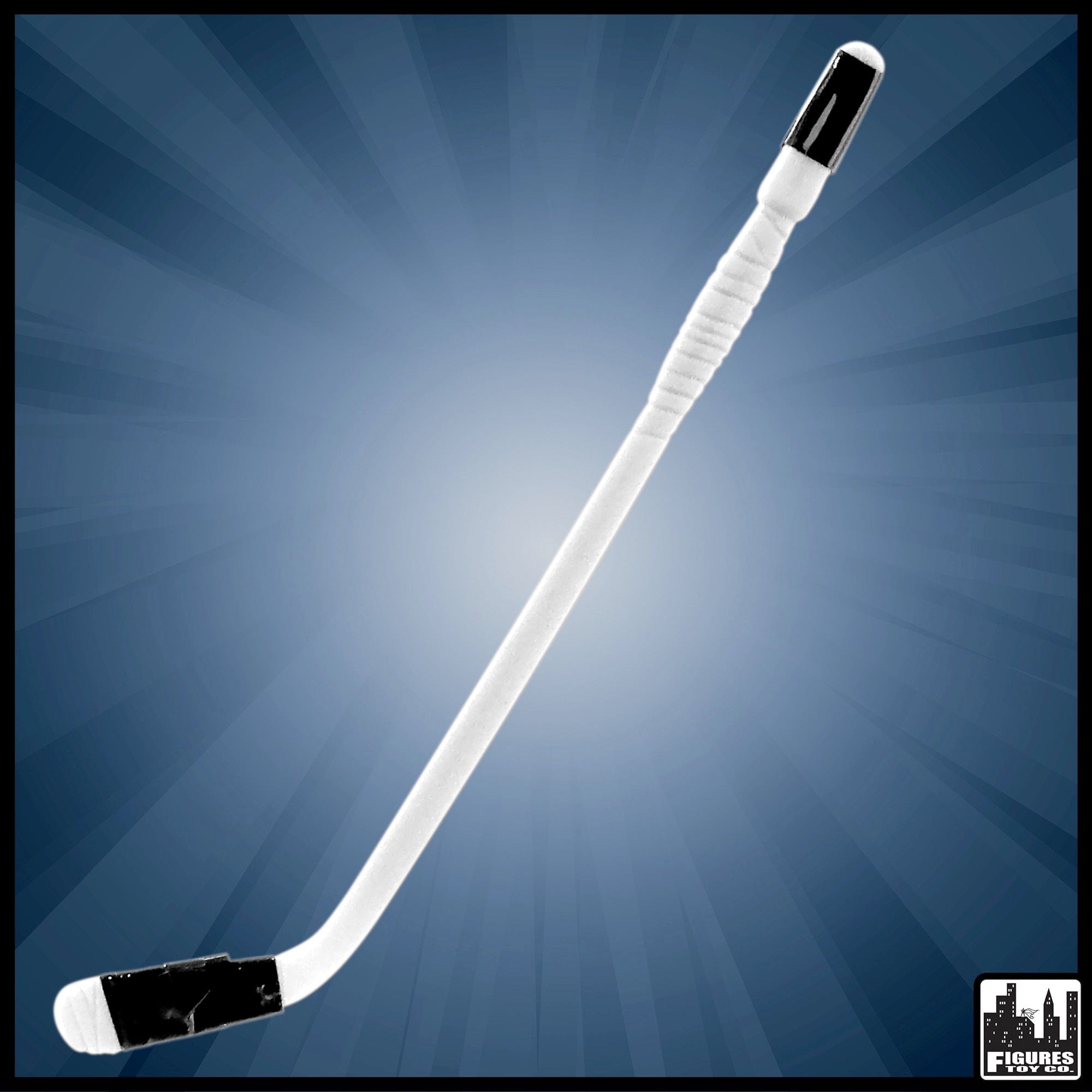The image depicts a digitally generated product shot with a predominantly blue background, featuring gradients of light and dark blue. The central element is a white ice hockey stick with a black-taped handle and a black-taped bottom. The stick is vertically oriented, with the curved end pointing towards the bottom left of the image. A radiant white light emanates from the center of the stick, blending into the blue background, giving the impression of light rays shining through. The image is framed by a black border and contains a logo in the bottom right corner. The logo, inside a black-bordered square, showcases a simplified cityscape with the text "Figures Toy Company" below it.